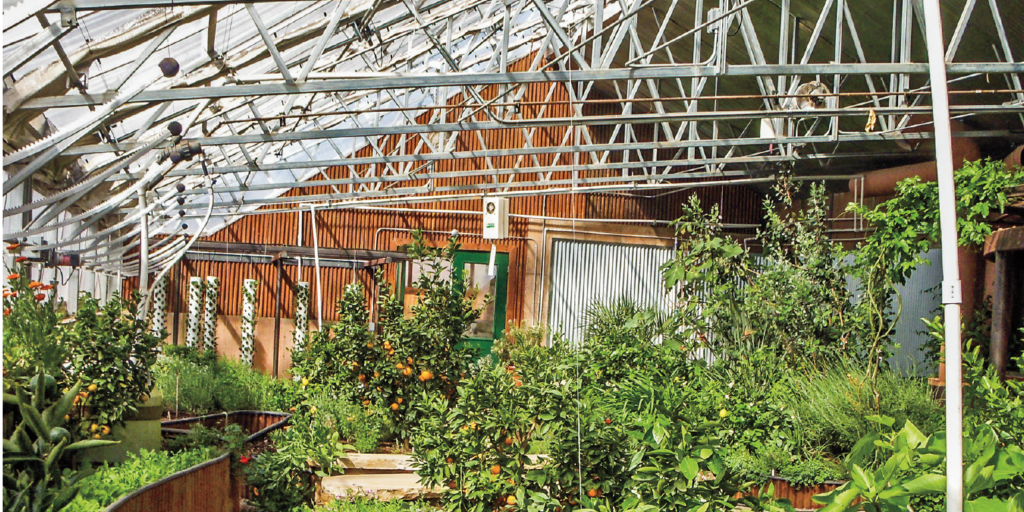This detailed color photograph captures the vibrant interior of a greenhouse structure, bathed in natural daylight streaming through its clear glass ceiling. The ceiling itself is reinforced with a network of crisscrossing metal beams, suggesting the presence of scaling mechanisms for maintenance. The greenhouse is lush with greenery, including an overgrown mass of shrubs, trees, and vines on the right, which is partially obscured by a variety of plants. 

On the left side, tiered wooden tubs host an assortment of plants, offering a glimpse of small fruits, possibly strawberries or other berries. In the background, there's a section of the greenhouse's brown siding, adorned with a green door that features a central window. Beside the door, a trellis of vines bears small orange fruits or flowers, adding a touch of color to the scene. Hanging white tubes with emerging green shoots dangle from the rafters, contributing to the dense foliage. Stone steps lead up to the area with the fruit-bearing plants, completing the picturesque and bustling greenhouse environment.